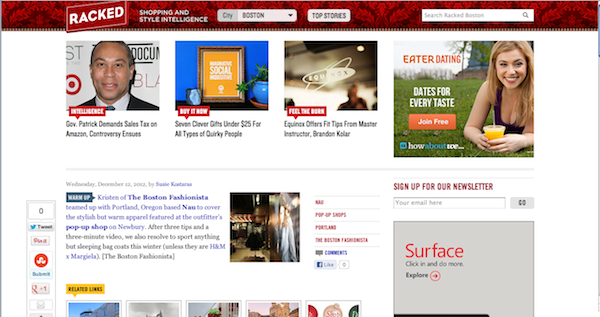The image displays the Racked Shopping and Style Intelligence website, tailored for the city of Boston. The interface features a prominent 'Top Stories' button and a search bar, allowing users to explore the Racked Boston site for specific content. 

The highlighted articles include:
- "Governor Patrick Demands Sales Tax on Amazon, Controversy Ensues"
- "7 Clever Gifts Under $25 for All Types of Quirky People"
- "Equinox Offers Fit Tips from Master Instructor Brandon Collar."

An advertisement promoting easier dating with the tagline "Dates for Every Taste" and a "Join Free" button appears, representing the brand 'How About We.' Additionally, there is a sign-up section for the website’s newsletter.

A Microsoft Surface ad is also visible. Below that, there are more articles, including one from Wednesday, December (year not specified). This article describes how Kristen from The Boston Fashionista teamed up with Portland, Oregon-based company to highlight the stylish yet warm apparel featured at the Outfitters pop-up shop on New Bern. It includes three tips and a three-minute video, advocating for alternatives to "sleeping bag coats" for winter wear.